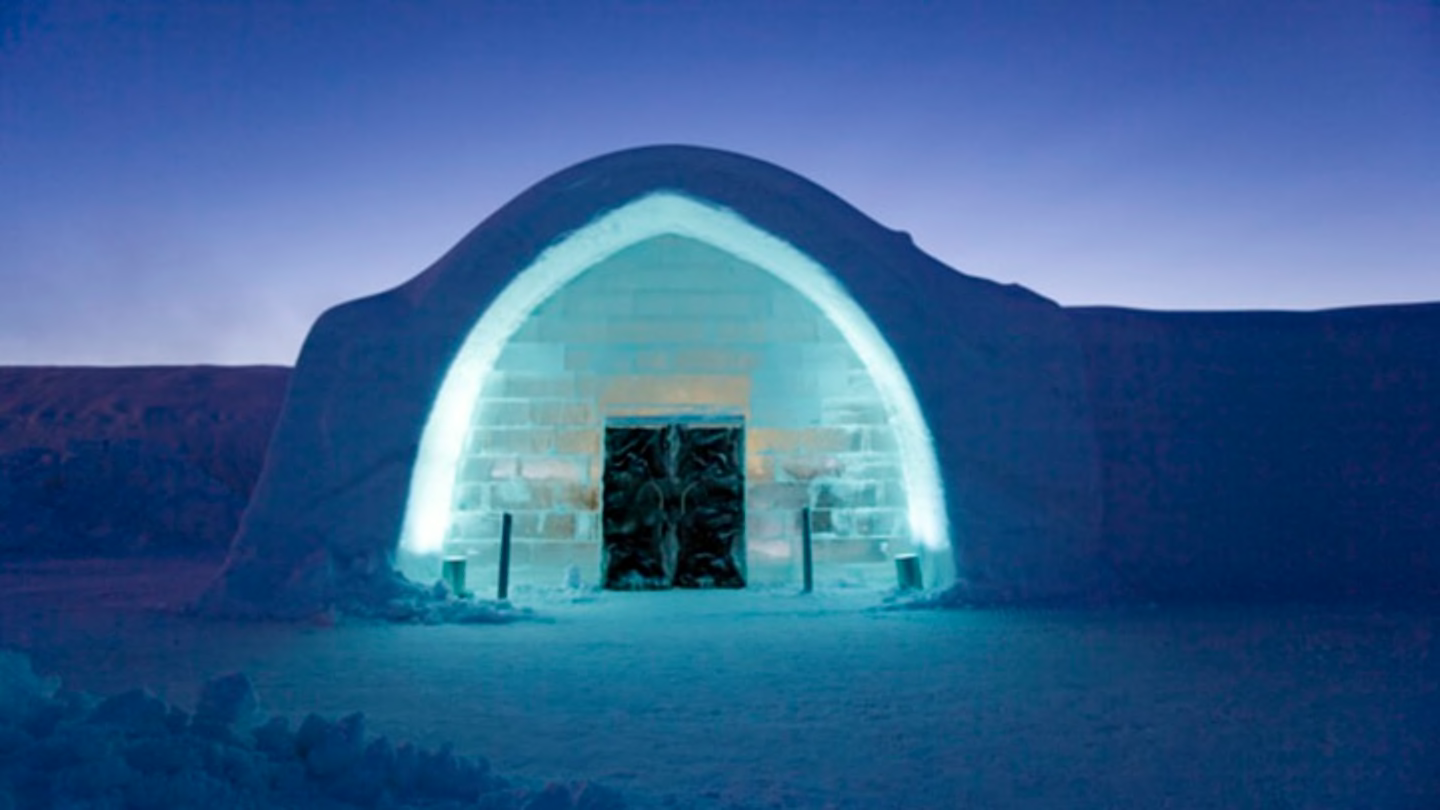The image features a mysterious structure set against a dark, bluish-purple night sky. The building, resembling an igloo or a rounded arch made of either ice or glass blocks, has a distinct entrance that appears black. An ethereal light outlines the top part of the arch, casting a glow on the front of the structure. Two large, round lights at the base of the arch flood the area with light, enhancing the building's icy appearance. The ground is laden with snow, accumulating in a pile on the bottom left corner and forming a wall-like structure on the right. In the background, a snow-covered hill adds to the wintry scene. Despite the overall darkness, a faint light peeks from behind the wall, hinting at a hidden source. The foreground includes discernible details like plants or rocks, adding texture to the otherwise monochromatic setting. The enigmatic image evokes a sense of cold and quiet isolation, with the snow and the unusual structure bathed in a surreal, bluish glow.